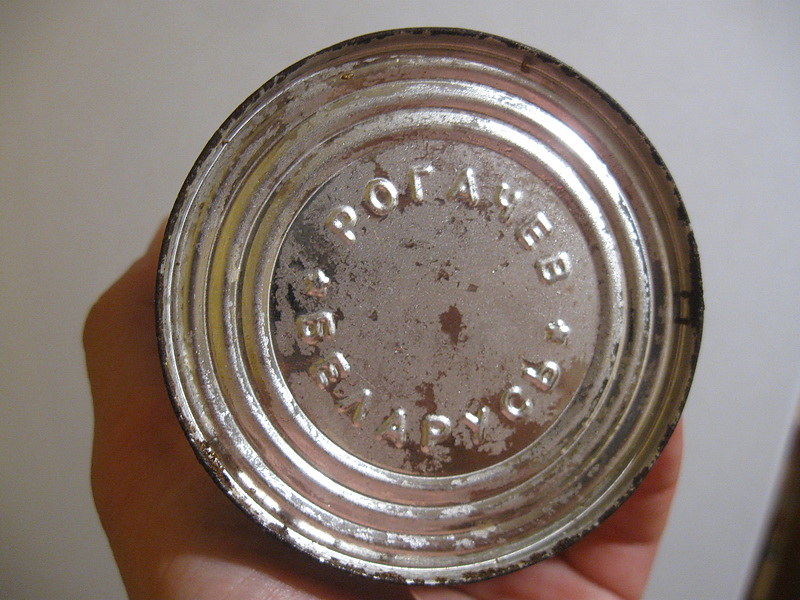This photograph captures a close-up view of a hand holding a can. Only a portion of the hand is visible, including parts of the palm, thumb, and pinky finger, gripping the can snugly. The top of the can faces the viewer, presenting a clear view of its aged, tarnished edges where a can opener would typically be used, suggesting a sense of antiquity. The aluminum surface of the can displays concentric rings, reinforcing its aged appearance. At the center of the can's top, partially legible text reads "P-O-T-A-N-E-E" at the uppermost point, hinting at the name of the product or company. The backdrop is a white wall, creating a stark contrast with the can and emphasizing its weathered condition. In the lower right-hand corner of the image, a dark triangular segment likely represents the edge of a countertop, subtly grounding the scene in a domestic setting.